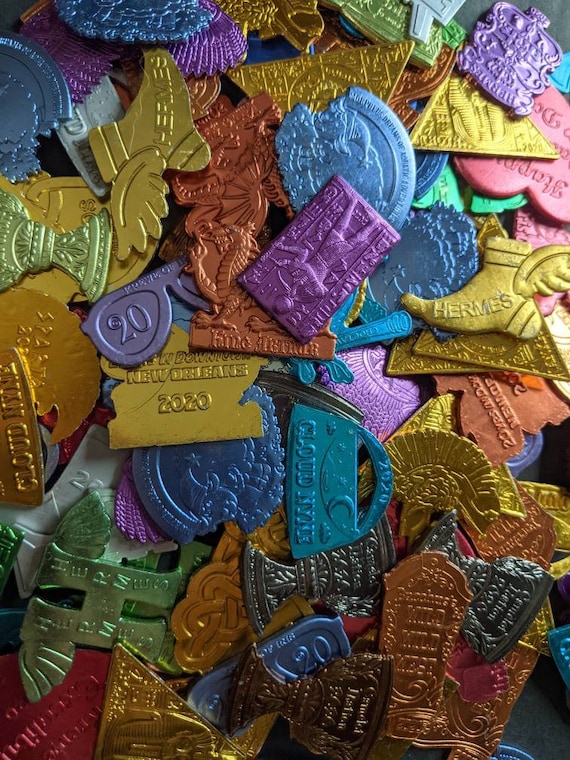This photograph captures a close-up of an eclectic assortment of colorful plastic trinkets traditionally thrown to spectators during Mardi Gras parades. The vibrant collection includes numerous small, shiny tokens resembling playful confetti, each inscribed with various words and images. Among the treasures are several shaped like the winged feet of Hermes or Mercury, emphasizing the mythological theme. A pair of sunglasses prominently displaying the year 2020 stands out amidst the chaos. The trinkets come in a spectrum of colors—gold, light blue, purple, orange, green, and steel—highlighting their diversity. Various shapes are identifiable, including pyramids, rectangles, suns, and even boots. Some tokens mention locations like "New Orleans" and "Wild Wild West," adding a geographical element to the display. The detailed, scattered arrangement invites closer inspection, revealing numerous Hermes tokens with distinct wing designs, all jumbled together to create a rich, textured tapestry of Mardi Gras festivity.